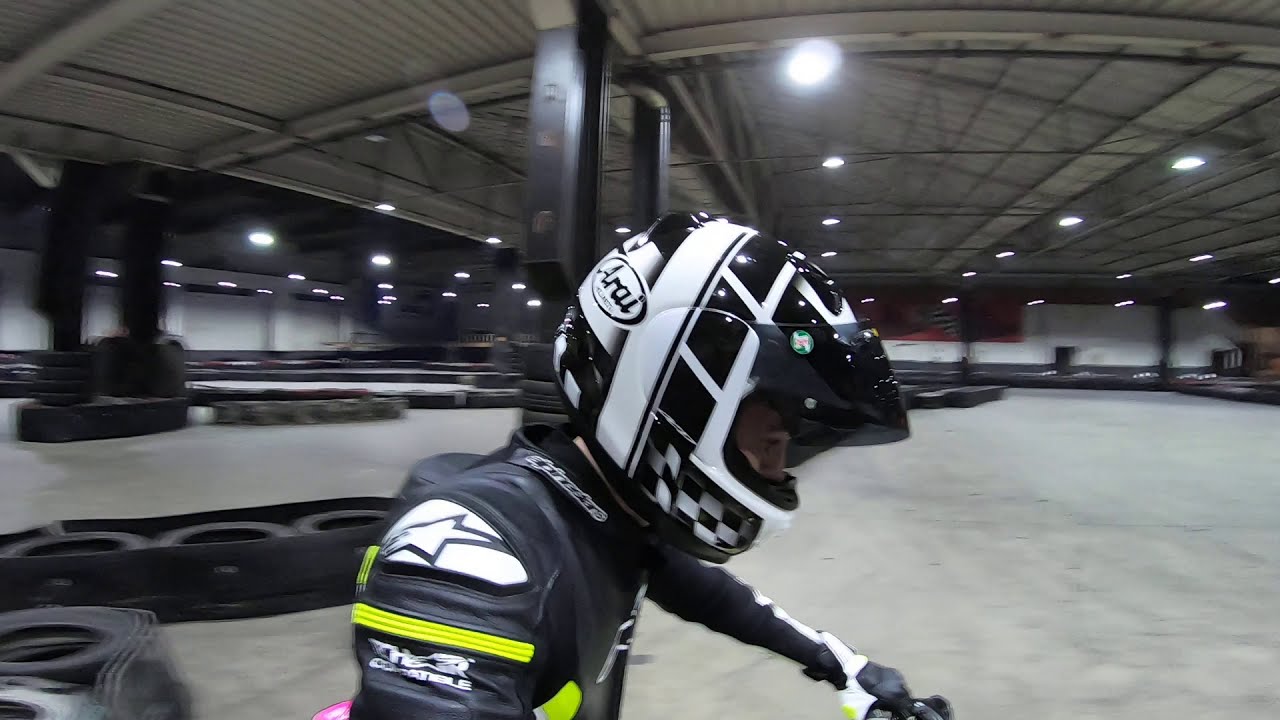In this detailed photograph, taken within a massive indoor arena, a motorcycle rider is prominently showcased close to the camera's lens. The photo captures the rider from shoulder level upwards, revealing a black and white Arai helmet and part of a black jacket embellished with striking bright green accents and white detailing, including a star on the shoulder. The rider, a white man, appears to be focused, likely practicing on a motorcycle, inferred by his left hand's position on an unseen handlebar. The expansive indoor space stretches out behind him, filled with tightly arranged tires forming racing barriers, situated on a vast cement floor beneath a high, corrugated ceiling supported by a network of rigging and metal rafters. The bright indoor lighting further illuminates the scene, emphasizing the disciplined setup of the track's boundaries.